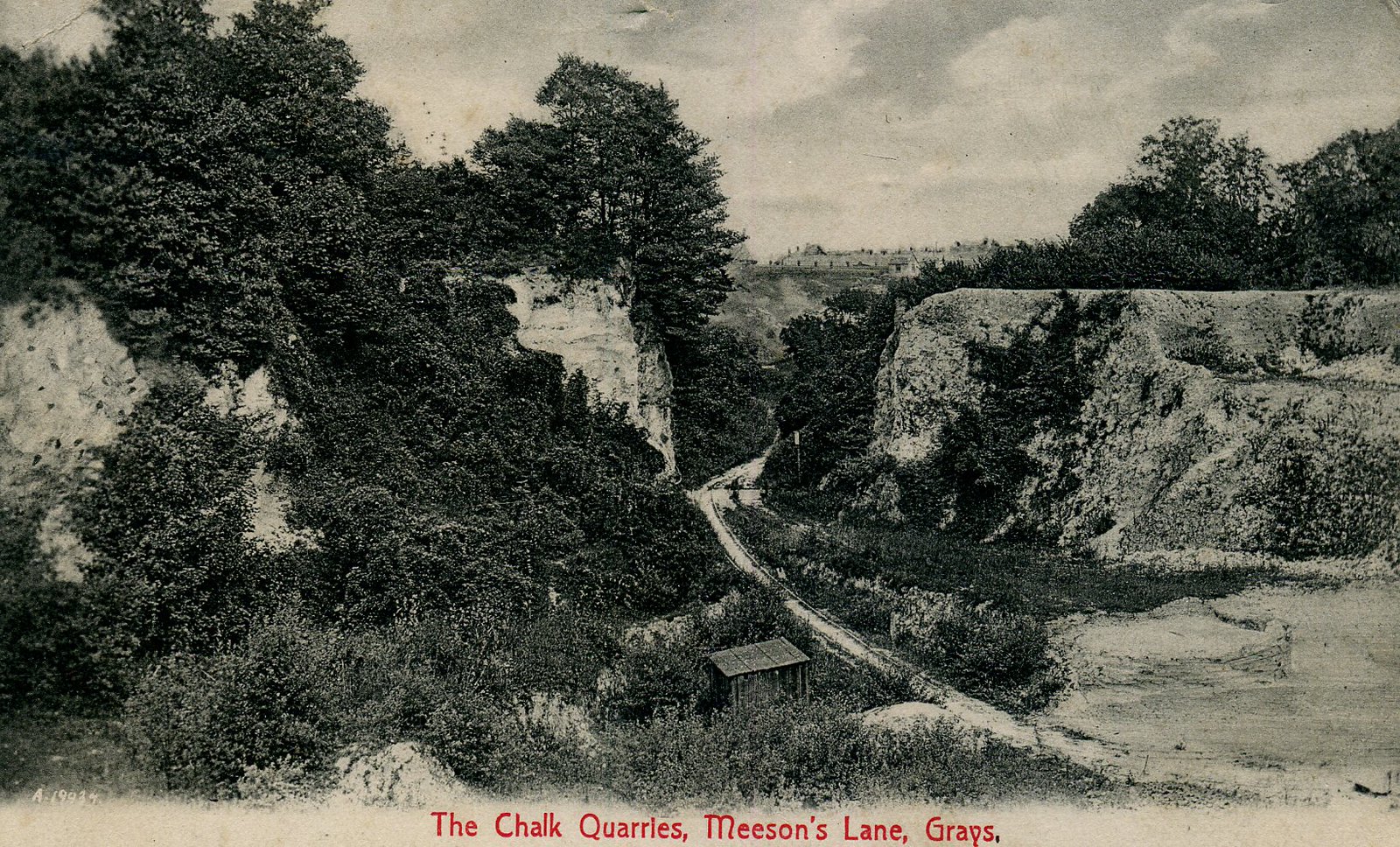This black and white photograph, seemingly from the 1920s or 1930s based on its condition and style, features the "Chalk Quarries, Mason's Lane, Grays," as indicated by the red text at the bottom. The image captures a dirt road winding between two prominent bluffs or hills, both swathed in trees and foliage. Each bluff's face is distinct, with the left cliff appearing white, likely indicating the chalk deposits. In the foreground stands a small wooden structure, possibly a shed or storage building, adding a touch of human presence to the otherwise natural setting. The road curves gently as it leads into the gorge, disappearing from view as it merges with the overgrowth and landscape. Distant structures, perhaps homes or other buildings, are faintly visible against a cloudy sky, which completes this serene yet industrially significant scene.